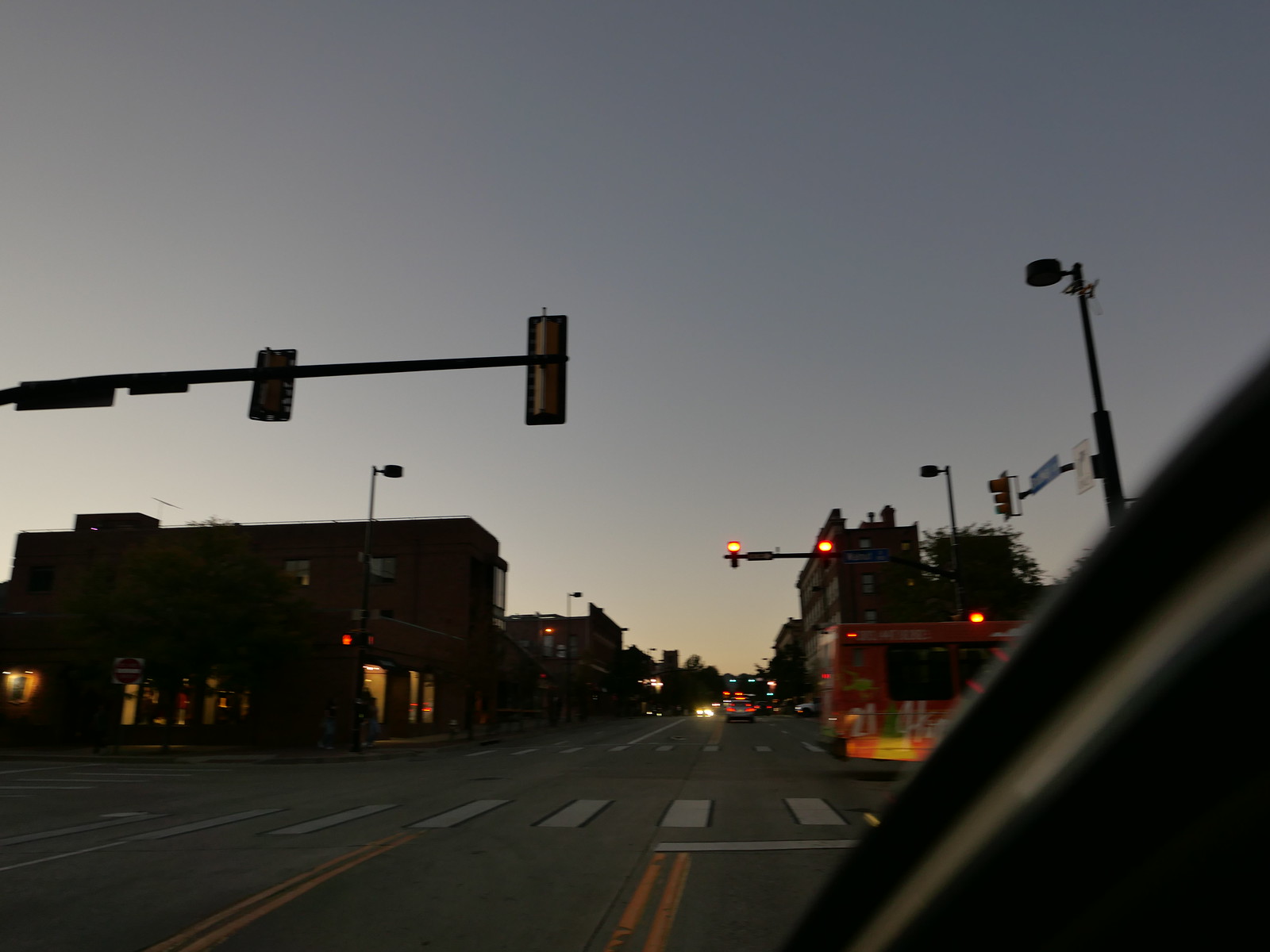A photograph captured from inside a car at sunset depicts a city intersection bathed in a dim, orange glow from the horizon. The image, taken through the car's window, shows the A-pillar of the vehicle in the lower right corner, indicating that the car is stopped at a red light. A red city bus is seen traveling across the intersection. The roadway, marked with yellow and white lines, extends into the distance, where headlights and brake lights from other vehicles are visible. Dark, silhouette-like buildings, possibly brick, line both sides of the street, with some windows illuminated. Trees can be seen in the far background, adding to the urban landscape.